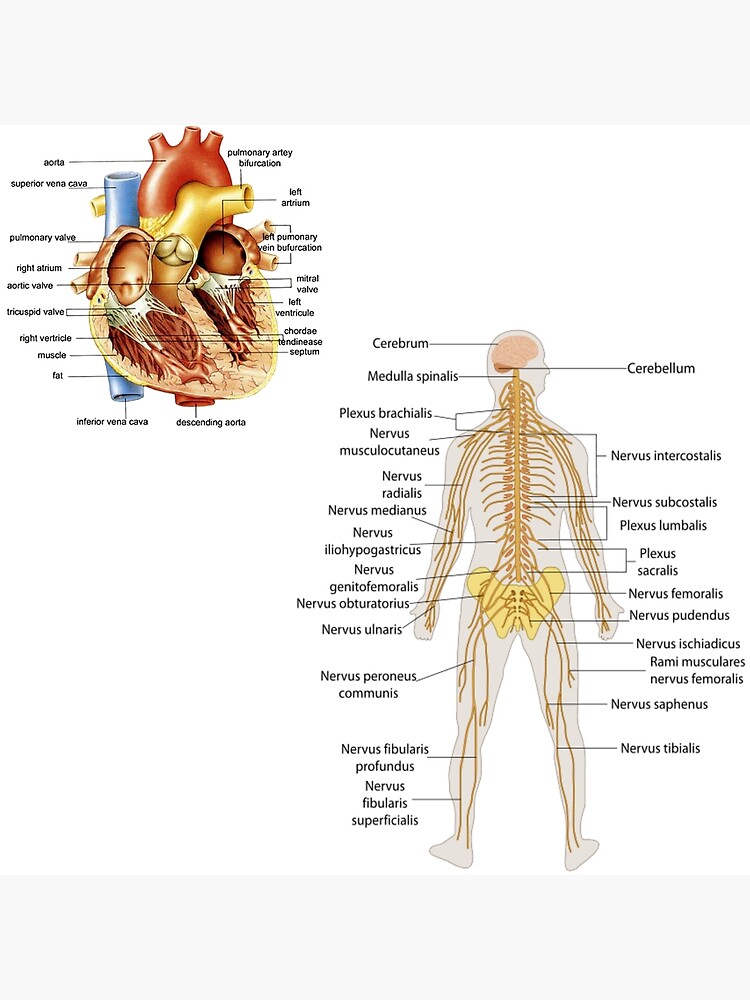This image features two detailed anatomical diagrams against a white background with light gray strips at the top and bottom. In the upper left corner, there is a colorful and labeled illustration of a cross-section of the human heart. The heart diagram highlights different areas, including the red aorta and blue superior vena cava, and is colored in hues of brown, yellow, red, and blue. The labels, marked in black text with lines pointing to specific parts, identify various veins, chambers, and structures of the heart.

In the bottom right corner, there is a detailed schematic of the human body focused on the nervous system. The diagram outlines the human body in light gray and shows the nerves in light brown, with the brain depicted in pink. Labels in black text identify parts from the cerebrum and cerebellum at the top to the nervus tibialis at the lower leg, with additional labeling of nerves and possibly some skeletal structures like the pelvic bones in yellow. This comprehensive presentation resembles illustrations typically found in medical textbooks, with each part meticulously identified to aid in learning the anatomy.